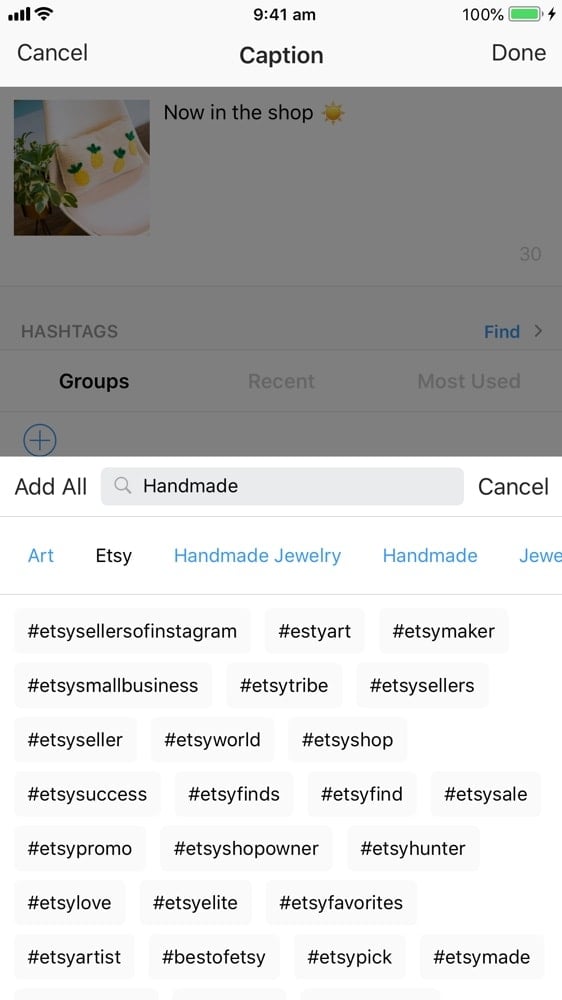### Detailed Description of a Mobile Screen Screenshot

The screenshot displays a mobile screen interface. Here's a detailed breakdown of the elements visible on the screen:

**Top Status Bar:**
- **Signal Strength**: Four out of four bars indicating full cellular signal.
- **Wi-Fi Connection**: Full bars showing a strong Wi-Fi connection.
- **Time**: Displayed in the middle, 9:41 AM.
- **Battery Status**: An icon showing the battery at 100%, with the icon colored green and a lightning bolt symbol indicating that the device is charging.

**Primary Action Bar:**
- **Left:** The word "Cancel" is visible.
- **Center:** A large space leading to the word "Caption".
- **Right:** The word "Done".

**Main Content Section:**
1. **Image and Caption Area:** 
   - At the very top of this section is a square image that appears to be a handmade product, possibly a bracelet or band. However, a transparent black overlay (approximately 80% opaque) makes it difficult to discern the details of the image.
   - To the right of the image, text reads "Now in the shop" accompanied by a star.
   - This section is likely part of a post on an app, possibly Etsy, given the context.

2. **Text Field**:
   - Below the image and text is a text field where the user might have entered a description or caption for the post. This section includes a thin line separator followed by an area for hashtags.

3. **Hashtag Area**:
   - A light gray section where hashtags can be added or viewed. Below this area are three columns labeled:
     - **Groups** (in bold)
     - **Recent**
     - **Most Used**

4. **Category and Hashtag Selection**:
   - Below another thin line separator, there are three elements:
     - A blue plus sign within a blue circle against a white background.
     - A search bar with the placeholder text "Handmade" and a "Cancel" button to its right.
     - A selection of categories, the current selection being "Etsy," with other categories like "Art", "Handmade Jewelry," and more.

5. **Hashtag Listings**:
   - The section beneath this is populated with around 50 light gray rounded-corner rectangles, each featuring different hashtags. Examples of the hashtags include "Etsy sellers of Instagram," "Etsy art," and "Etsy maker." The hashtags seem related to Etsy and are displayed on a white background.

This detailed description provides a comprehensive view of the various elements on the screenshot, encompassing both the interface and the content within it.